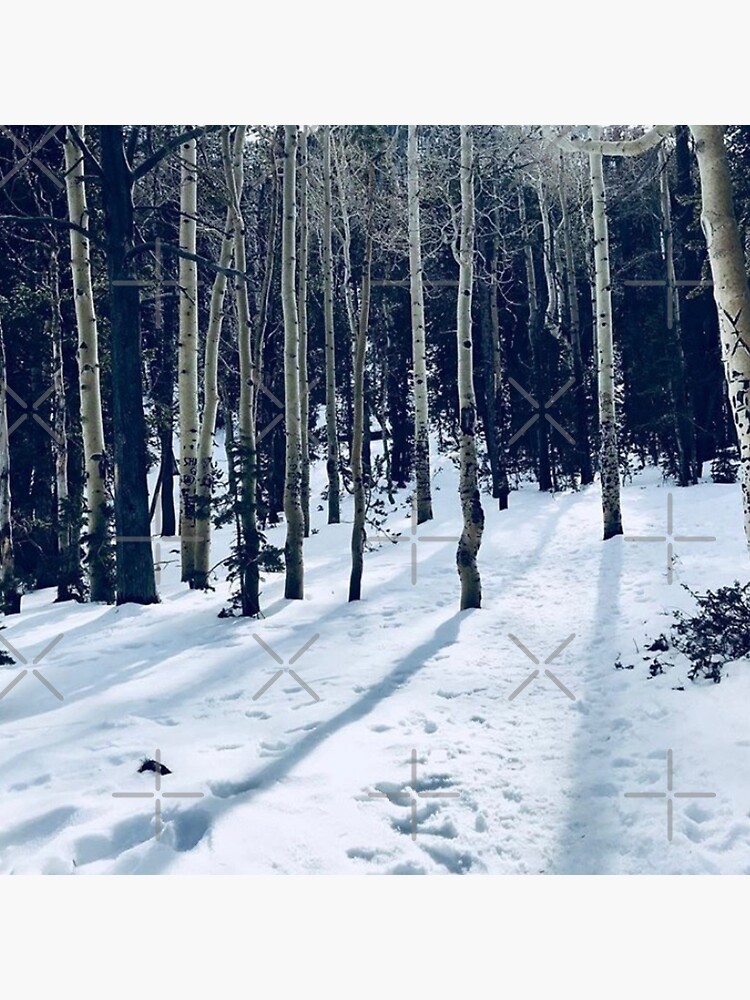This photograph captures a serene wintery scene in a forest. The foreground is a snow-covered clearing, featuring tracks that lead towards a dense tree line just several feet away. The snow appears fairly thick, interspersed with low shrubs poking through. Bare trees dominate the scene, their tall, slim trunks rising without limbs on the lower portions and bearing branches high up without leaves. Distinctively, birch trees with their smooth, white bark stand out at the forefront of the tree line, mingled with other gray and black-hued trees. The only greenery present comes from a few evergreen trees. Despite the lack of color, the detailed textures suggest it might be a black-and-white photograph. Superimposed on the image are three large X's and three plus signs, creating a graph-like overlay.